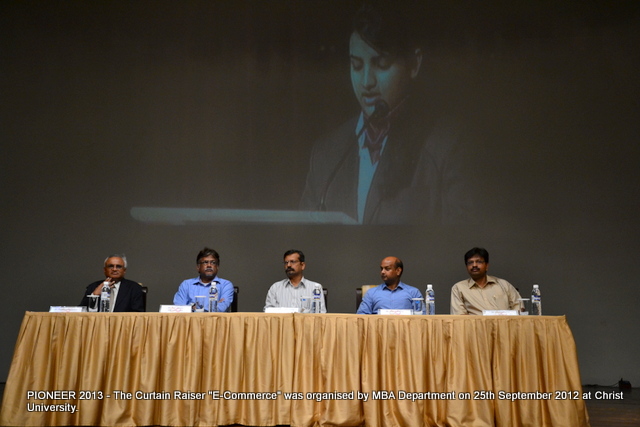The image depicts a panel discussion at a conference, held indoors at Christ University on 25th September 2012, organized by the MBA Department. The event is titled "Pioneer 2013: The Curtain Raiser - E-commerce," as indicated by the white text running along the bottom of the photo. Seated at a long table draped with a golden cloth are five middle-aged men, likely of Indian descent. From left to right: the first man wears a grey suit and has white hair; the second man, darker-skinned, wears a blue shirt and glasses; the central figure sports a light-striped shirt and has a black mustache; next is a shorter, bald man in a blue shirt; and on the far right, a man with bushy black hair, mustache, and tan shirt. Each has a bottle of water and a white name placard in front of them. Behind the panelists, a large screen projects the image of a young woman, likely the presenter, dressed in a suit jacket and scarf, her eyes downcast as she speaks into a microphone at a podium.